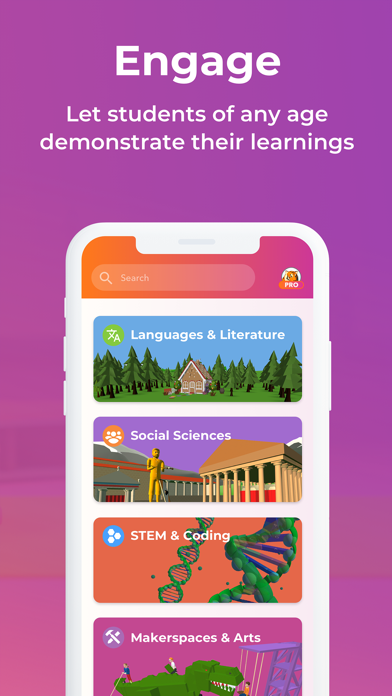The image is a screenshot of a mobile device displaying a vibrant, colorful interface set against a pink background. On the screen, there is a graphic of a mobile phone with four distinct images. The top image depicts a house under clear blue skies surrounded by green trees, with the text "Languages and Literature" written in white. Below that, the second image features a stylized human silhouette on a purple background. The third image displays green DNA strands against an orange backdrop. At the very top, the main image features the caption in white text: "Engage, let students of any age demonstrate their learnings." The detail and richness impart a dynamic and educational vibe, highlighting various learning disciplines and encouraging interactive engagement.